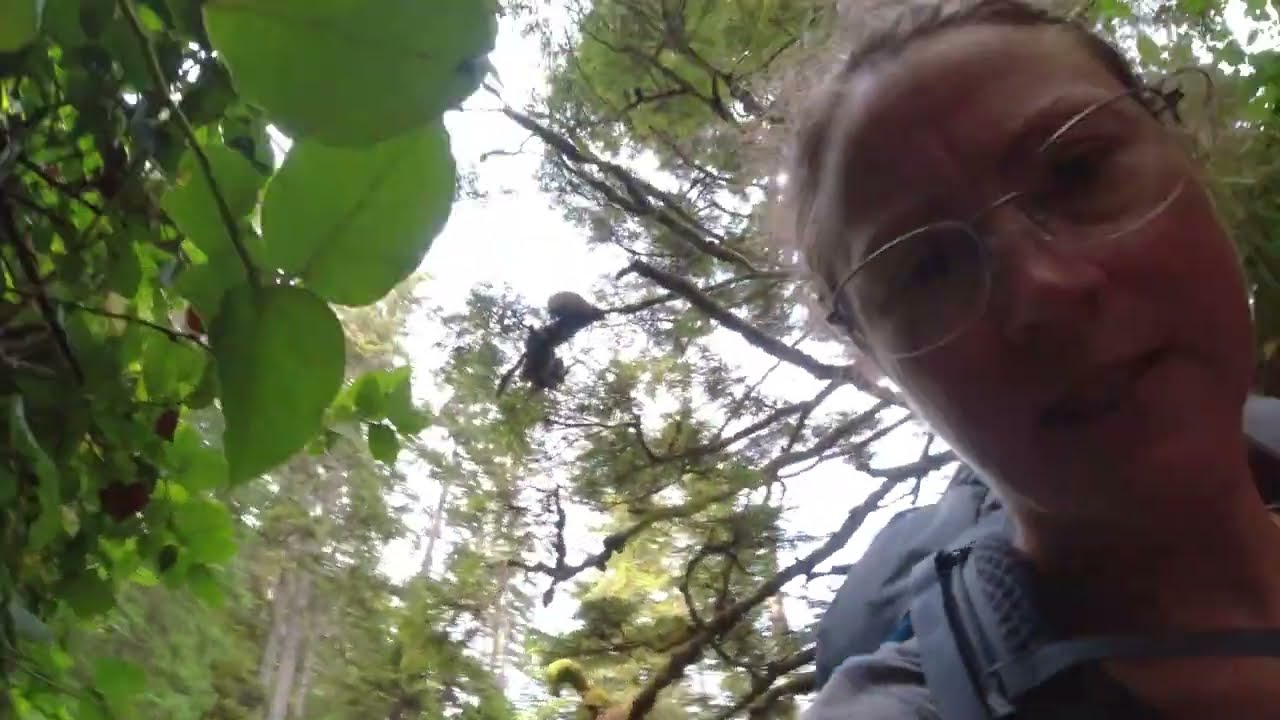The image captures a close-up of a woman’s face, occupying the right third of the frame. Her head is tilted slightly, and she wears glasses, her light brown or dirty blonde hair pulled back. The woman, in her thirties, is dressed in a blue coat and carries a grey backpack on her shoulder, suggesting she might be hiking. Her expression is somewhat curious, with scrunched eyes and a half-open mouth, as she looks directly at the camera. The lighting is dark, casting shadows on her face which makes fine details less discernible. She stands amidst a forest setting with a mix of green and brown trees around her. The sky above is overexposed, appearing white, while the middle of the image presents a burst of light streaming through the tree branches. The left third of the frame is dominated by large leaves and dense branches, blocking much of the light and casting further shadows, while the background reveals taller trees or possibly a cliff face.